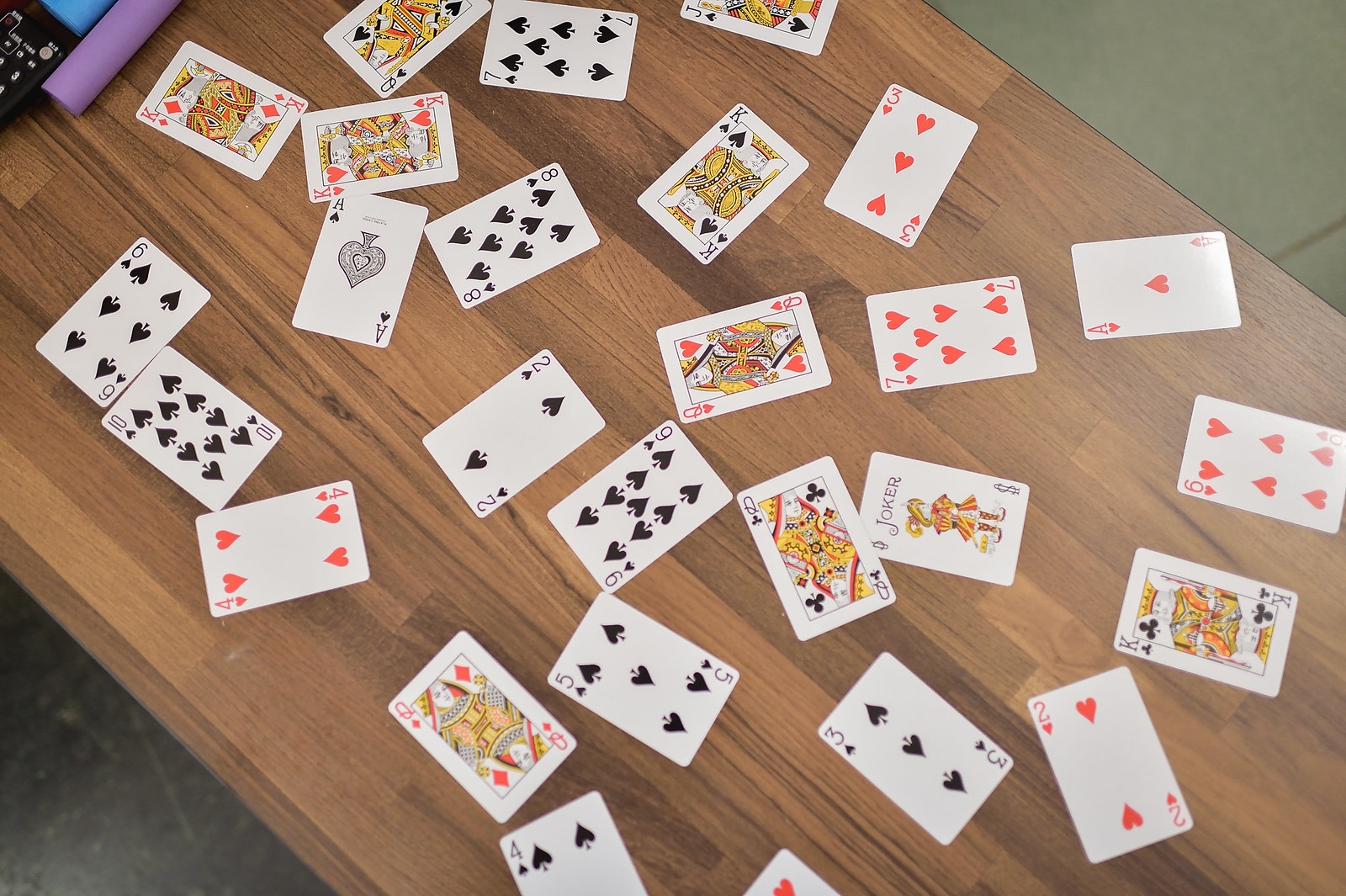In this photograph, we're looking straight down at a tabletop with a woodgrain finish. Scattered across the table are numerous face-up playing cards, barely touching each other. Among the cards, there are all four kings, all four queens, and a single jack. Various suits are represented, with a noticeable number of spades, including an ace, a two, a three, a five, a nine, a six, and a ten. In the hearts suit, you can spot an ace, a two, a three, a six, and a seven. There is also a joker card present. The cards are spread out fairly evenly but lie at different angles. In the far upper left of the picture, there's a rolled-up purple item that looks like a stick, along with a black object featuring white markings, likely part of a TV remote control given the visibility of numbers. Above this is a small, visible corner of a blue object.